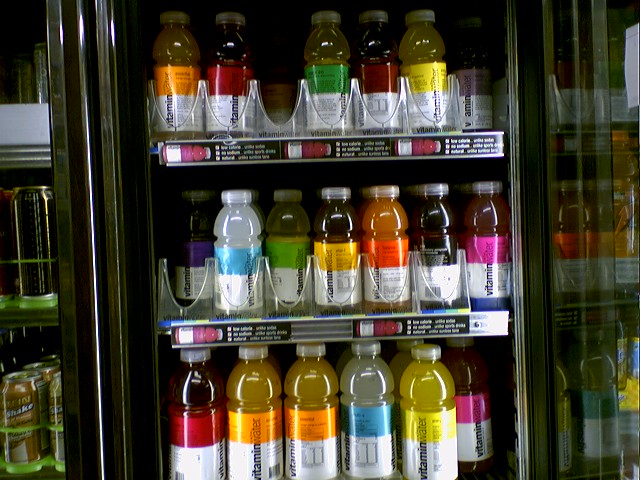This image captures a heavily stocked drink cooler found in a gas station or convenience store, prominently displaying a variety of Vitamin Water bottles. The cooler door is open, hinging to the right, and revealing multiple shelves lined with the colorful beverages. The top shelf features smaller bottles with labels in colors such as orange, red, green, and yellow, while the middle shelf holds bottles with white, light yellow, orange, purple, and red labels. The bottom shelf, dedicated to the larger bottles, showcases a progression of red, yellow or orange, clear, yellow, and another red bottle. Some sections have noticeable gaps where bottles have sold out, indicating the popularity of particular flavors. The right side of the scene includes a reflective surface, making it challenging to discern the details of the beverages in that part of the cooler. Additionally, a couple of cans are visible on the left side, with one appearing to have the word "shake" on it, although details are unclear. The vibrant array of Vitamin Water labels includes colors like green, red, blue, yellow, orange, pink, purple, black, and white, set against mostly white lower halves of the labels, all emblazoned with the brand name.